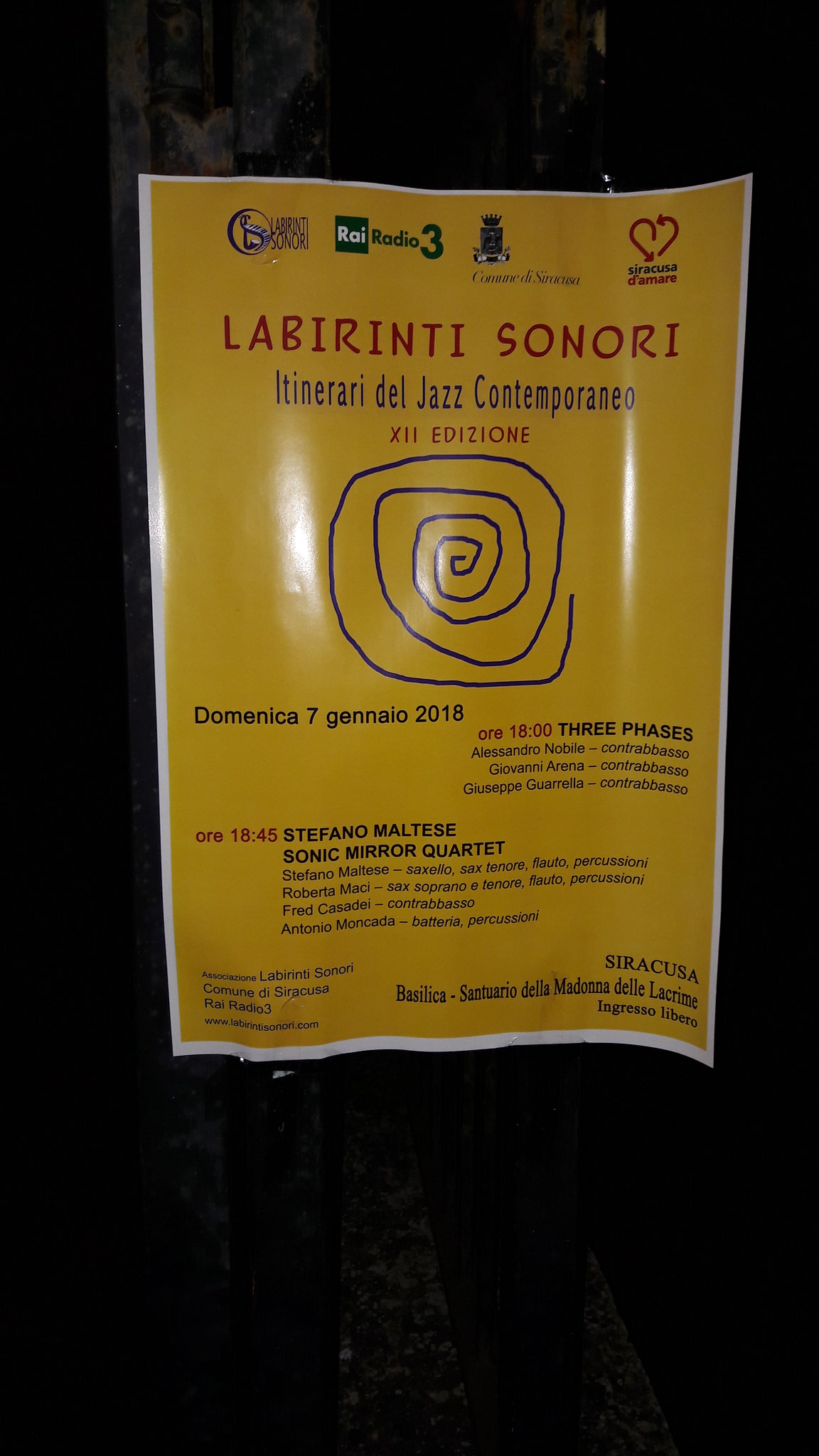The image features a yellow poster taped to a wall or signpost, likely captured at night given the dark background. Dominating the top portion of the poster are four sponsorship logos. Below the logos, a large red headline reads "Labyrinthi Sonori," with the phrase "Itinerari del Jazz Contemporaneo" in smaller blue text underneath, indicating a contemporary jazz event. It highlights that this is the "XII Edizione," or 12th edition. The center of the poster showcases a hand-drawn, jagged spiral resembling a Peruvian symbol. Event details include the date "Domenica 7 Gennaio 2018" and a performance by "Stefano Maltese Sonic Mirror Quartet" noted in black text. Other inscriptions include "three phases," and additional information outlined in various colors. The bottom of the poster bears the name "Syracuse."